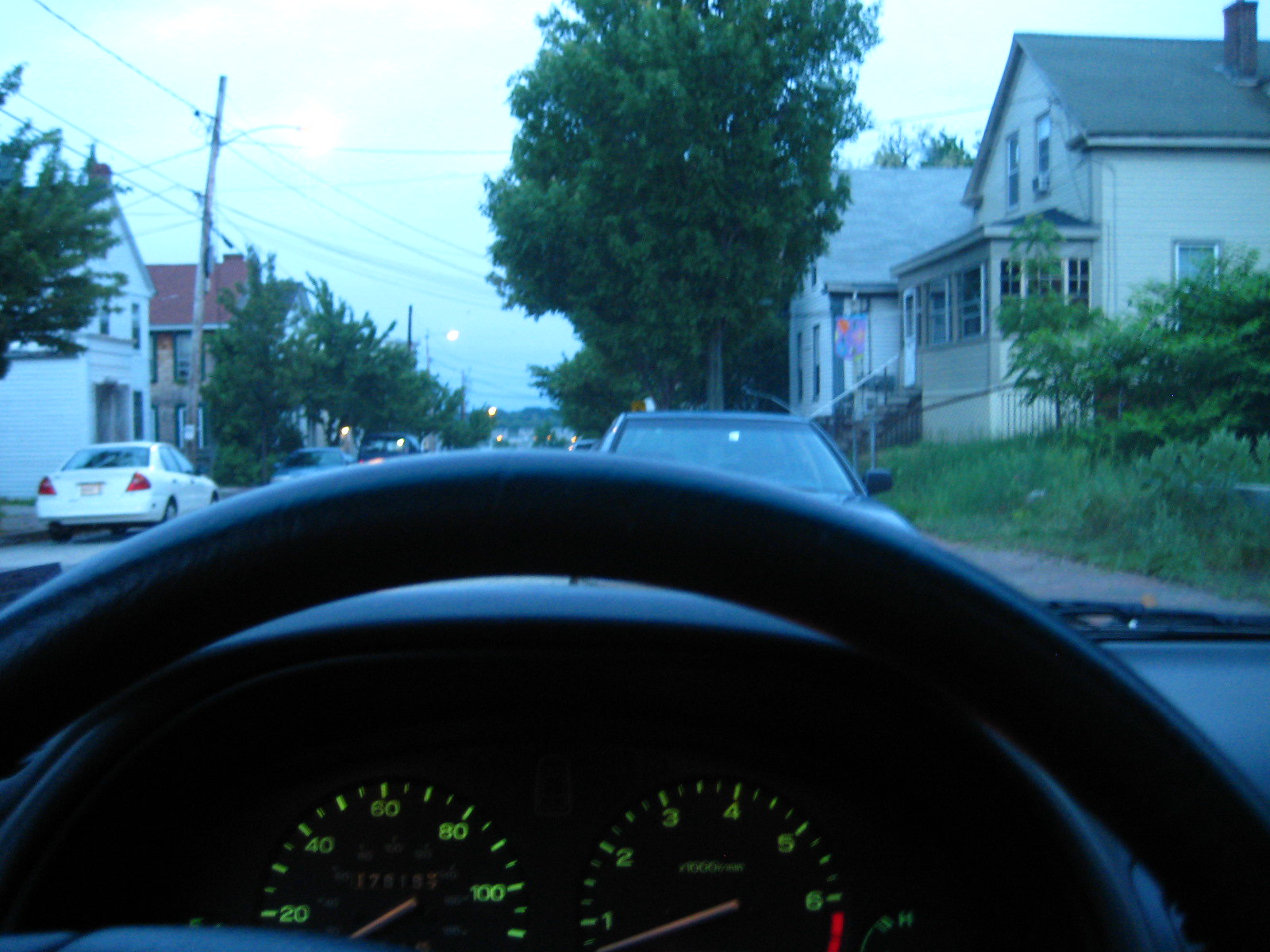This photograph captures the perspective from inside a car, focusing on the driver's view. The lower half of the image prominently displays the car's dashboard and steering wheel, with green-lit gauges indicating the speedometer and RPMs. Through the front window, a residential street comes into clear view. Houses of a white or whitish hue line both sides of the street, along with cars parked in front of them. Vegetation, including green trees, adds a touch of nature to the scene, while sidewalks accompany the roadway. Overhead, power poles and electric power lines crisscross the sky, and the moon is faintly visible, adding a serene touch to the landscape.